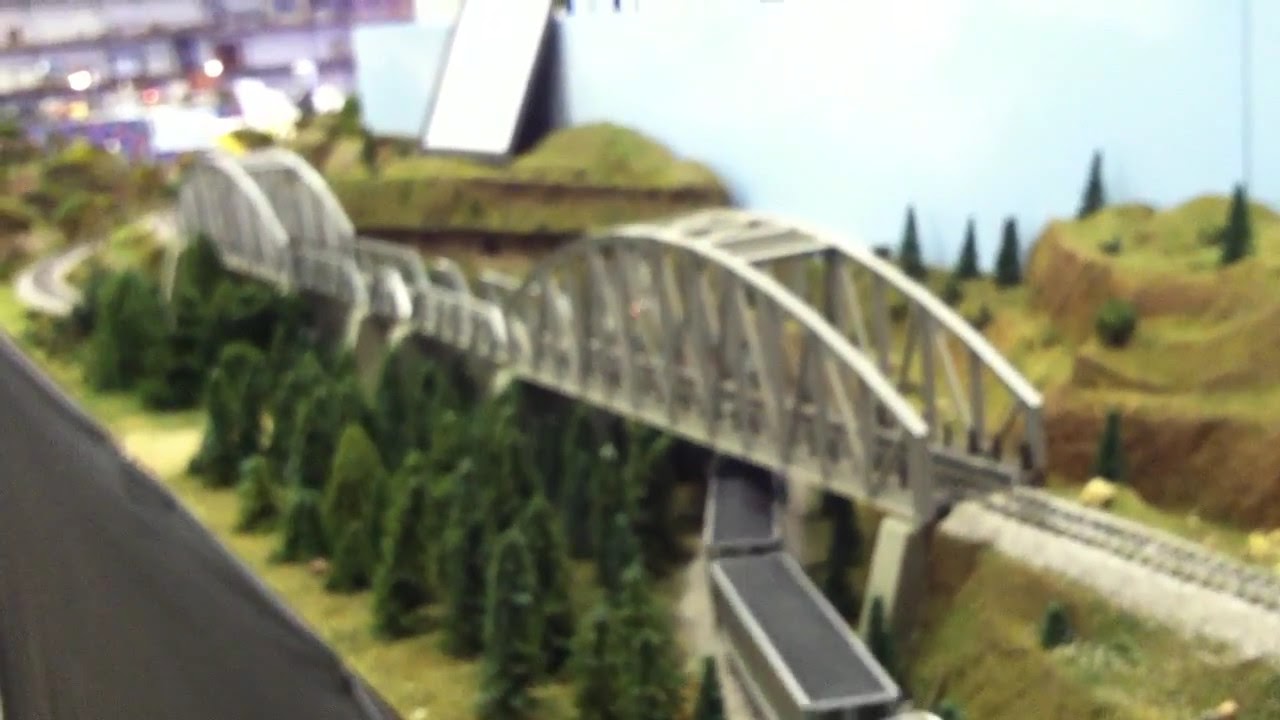The image is a grainy, blurry photograph depicting a miniature model landscape with a railway bridge. The grey railway bridge extends from the lower right to the upper left, and is designed for a model train. Underneath the bridge, you can see numerous green pine trees. The backdrop features a blue board representing a light blue sky, and some mountains are faintly visible behind the bridge. The train itself appears to be covered in mossy paint and is moving along the tracks in the lower right section of the image. Wagons or train cars are also visible passing below the bridge. The overall scene resembles an animated video game due to its miniature scale and low-resolution quality.